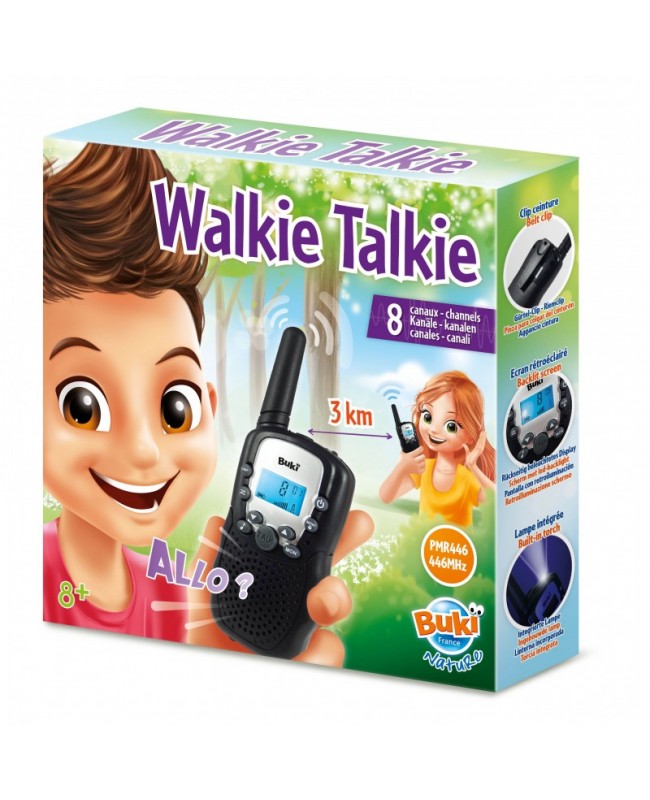The image showcases a well-detailed, 3D-angled product box for walkie-talkies, prominently displaying all three dimensions. Set against an all-white background, the box reveals various informative elements. Central to the cover are cartoon illustrations of a boy in a red shirt and a girl in a yellow shirt; both are actively using black and silver walkie-talkies. The boy, positioned in the foreground, holds the walkie-talkie in his left hand, while the girl in the background listens with the device to her ear. Between them, an orange double-headed arrow indicates a range of 3 kilometers.

The packaging features vibrant colors including purple, white, green, brown, yellow, and orange, giving it a toy-like appearance. The text "walkie-talkie" is emblazoned in large purple letters with a white outline. Above the girl, more purple text on the background highlights "8 channels" in multiple languages (including "canale" and "canalan"), indicating the box is not primarily in English. Additional details include "PMR 446, 446 megahertz" written in purple, alongside the word "aloe." The box is adorned with various logos and small textual elements providing further product specifications. The setting of this box shot appears outdoors with a grassy backdrop, trees, and a blue sky visible.